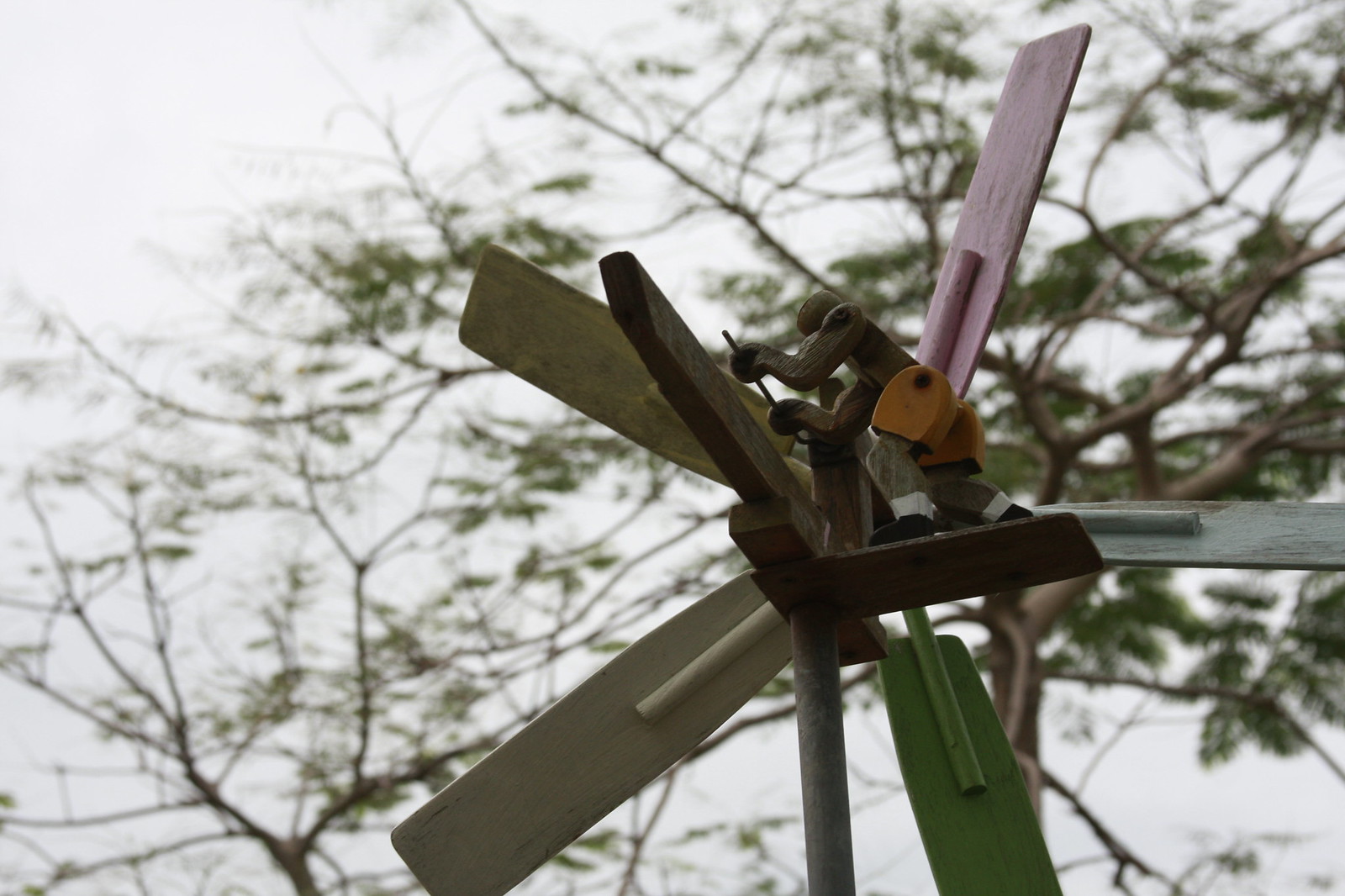The image depicts a curious structure resembling a windmill with a wooden figure perched on top. This windmill features five colorful blades—two are grayish-silver, one light purple, one brown, and one dark green. The wooden figure has the appearance of a person engaged in an activity, possibly rowing or turning a lever, perhaps to imply movement of the windmill’s blades. The figure is adorned with a green jacket and a blue-strapped kit, holding a stick, possibly engaged in a repair task. The background illustrates a light sky, with sparse branches bearing a few green leaves, hinting at the turn of the season, possibly winter. The entire scene is set outdoors, likely on a street with a large, near-bare tree suggesting the colder season.